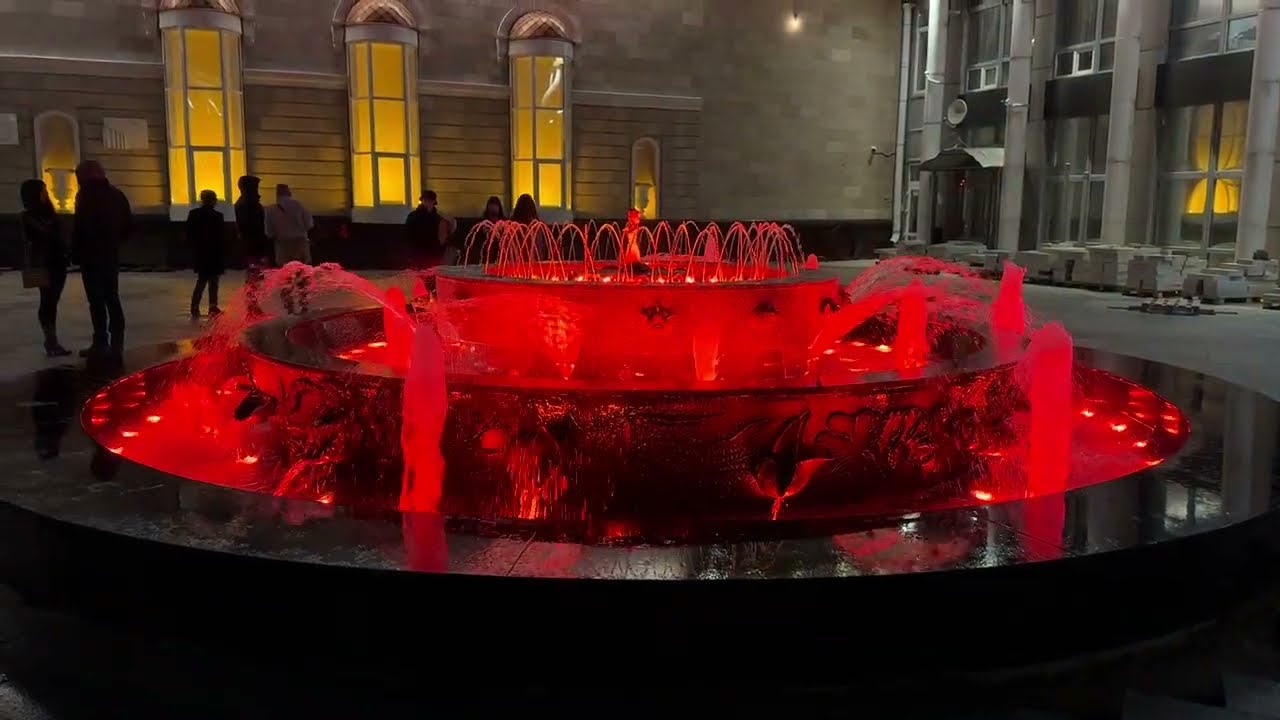This image is a color photograph taken at night in landscape orientation. The central focus of the image is a large, circular, multi-tiered fountain, prominently illuminated with red lighting. The fountain, which spans the width of the frame, features several spouts of water cascading upward from its three distinct tiers, all bathed in a vibrant red glow. Its base appears to be constructed of black marble, enhancing the vivid lighting effect.

In the background, two large buildings frame the fountain. To the left, a tall structure with three immense, yellow-lit windows and dome canopies stands prominent. The building to the right is characterized by four substantial columns and includes floor-to-ceiling windows, one of which is also illuminated in yellow. This building extends at a right angle, connecting with the second building. The setting appears to be an entertainment or cultural complex, possibly a concert hall or theater.

Several people, about a dozen, can be seen walking or gathering in the courtyard behind the fountain, adding a sense of liveliness and scale to the scene. The detailed realism of the photograph captures the elaborate and dynamic interplay of light, water, and architectural elements, creating a striking nocturnal cityscape.